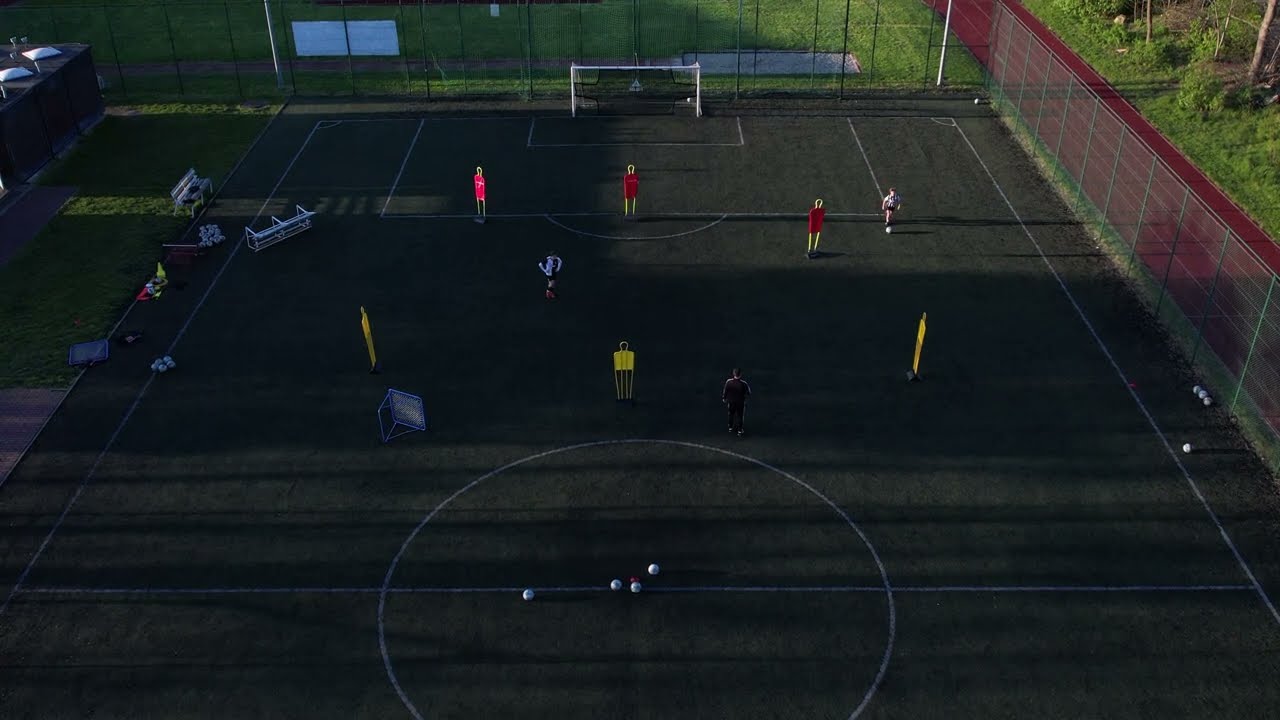This image depicts an aerial view of a fenced-in soccer field designed for practice. The scene includes a couple of real individuals and several mannequins or training dummies dressed in red and yellow, placed strategically around the field. Four soccer balls are neatly positioned at the midfield line within the larger white circle marking the area. The field itself features a dark, grayish-green surface marked with white lines. Dominating the northern part of the field is a white goalpost. Surrounding the soccer field is a tall chain-link fence, and to the far right, a red pathway is visible outside the facility. The entire setting is observed from an elevated angle, providing a comprehensive view that highlights various colors like dark green, light green, red, gray, black, blue, and yellow. The elevated perspective also reveals surrounding grass areas and additional practice equipment like cones scattered about.